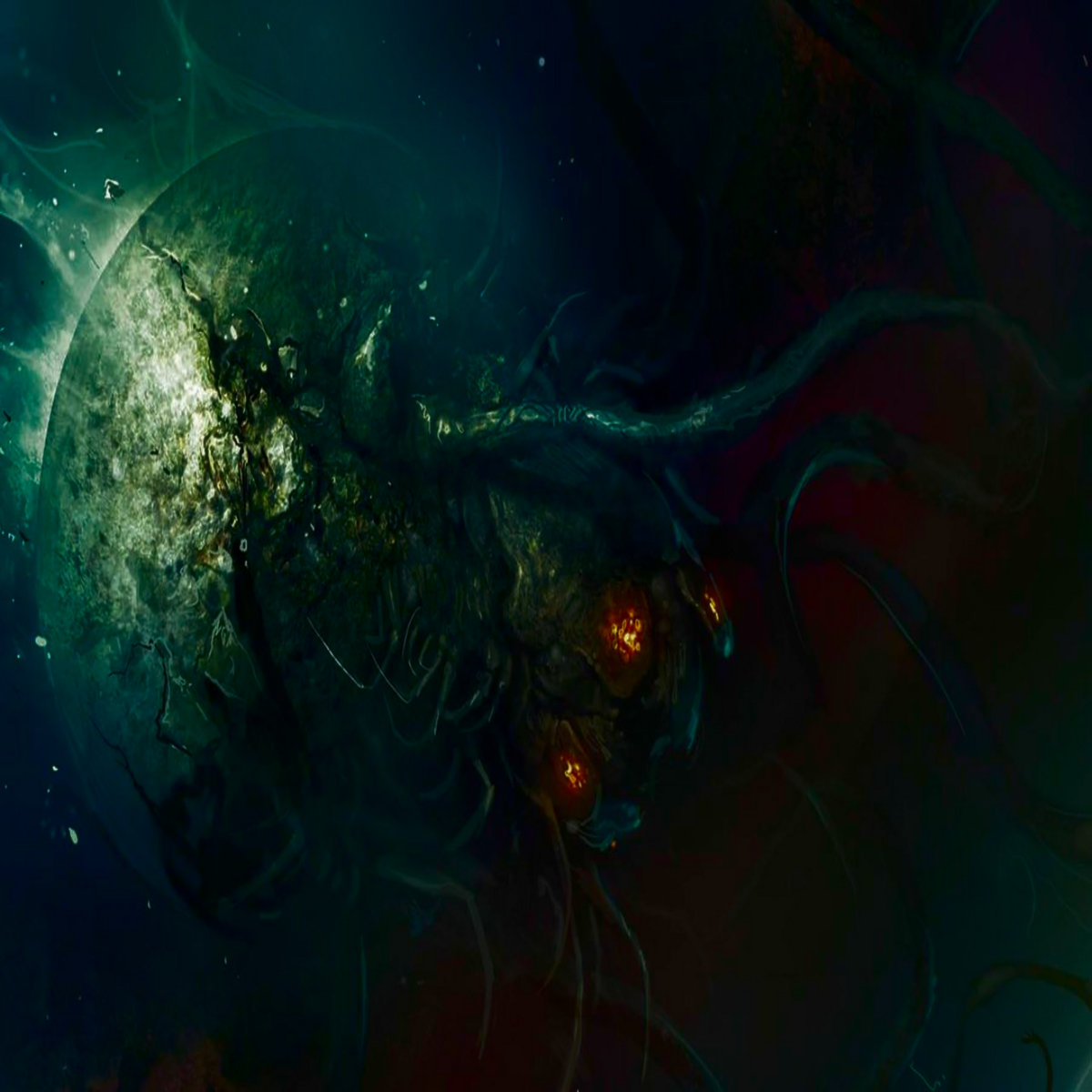The image appears to be an artistic rendition of an alien creature set against the backdrop of outer space. The central figure resembles a science fiction sea creature, characterized by a round body with several tentacles extending from its face area. Its most striking feature is the presence of three glowing orange eyes that pierce through the darkness. The creature itself seems to be emerging from or bursting out of a gelatinous, greenish-yellow substance, which adds to its otherworldly appearance. Surrounding the creature, the setting is rich with details—a sky filled with blue tones and scattered stars, hinting at the vastness of space. In the background, a lighter, curved element suggests an explosion or impact. Additional nuances, such as barely visible reddish-orange lights, contribute to the mysterious ambiance, further cementing the scene's science fiction motif.